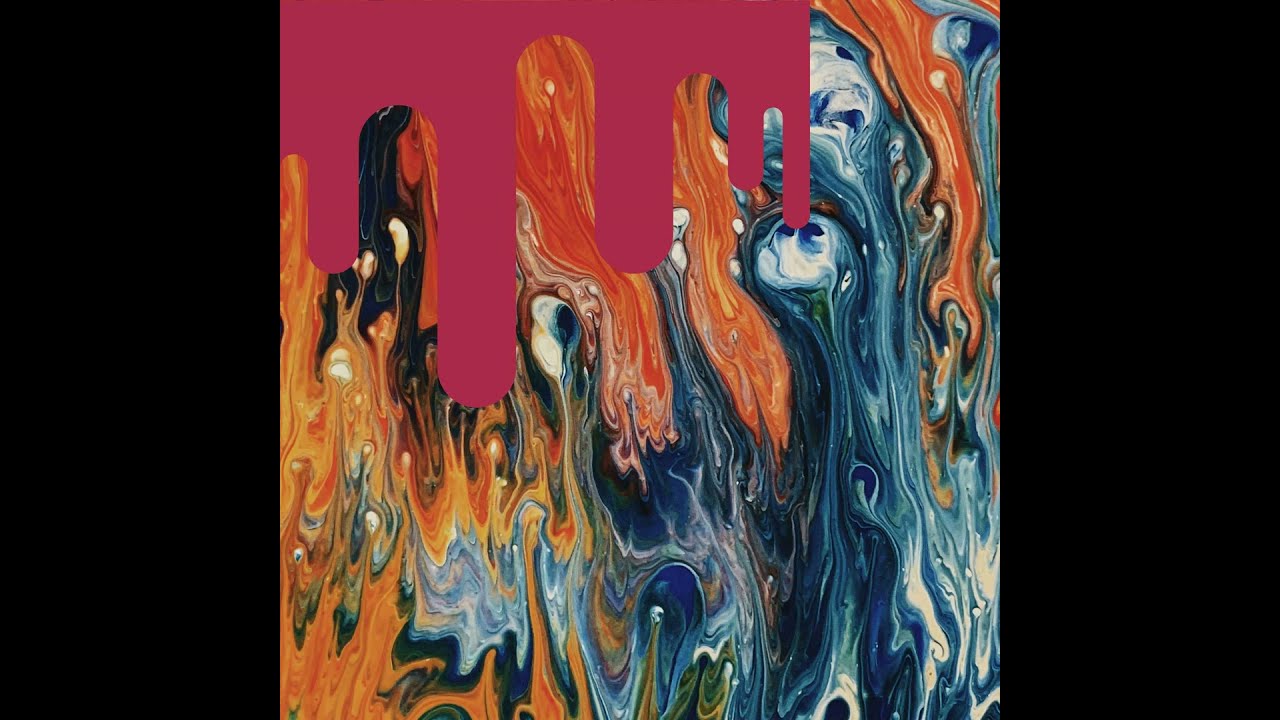The image is a piece of abstract art, potentially both digitally created or hand-painted, embodying a psychedelic aesthetic with vibrant, intermixing colors. At the center of the image, the colors create a dynamic and marbled texture, resembling wax dripping upward—perhaps an illusion created by flipping an original downward drip. The color palette features a spectrum including black, red, orange, yellow, various shades of blue, white, green, and silver, alongside light blue, and dark blue, giving it a fiery, lava-like appearance. The border on both the left and right sides is a solid black, drawing focus to the intricate painting within. Amidst the swirling colors, one can discern an almost anthropomorphic form in the middle: two eyes formed from blue and white, surrounded by orange, giving the impression of a face looking up to the sky. This sky transitions to a purple hue, enhancing the cascading effect of the vibrant wax-like patterns. With no text present, the painting’s central position invites viewers to immerse in its flowing, mesmeric design.